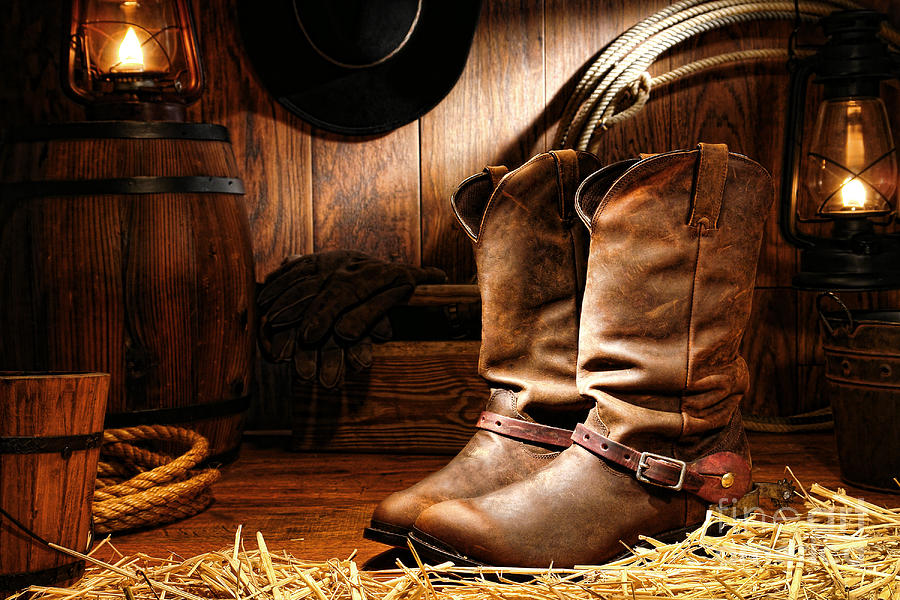This highly detailed still life photograph emphasizes a pair of new, brown leather cowboy boots, adorned with reddish-brown ankle straps with buckles. The boots are prominently positioned slightly towards the bottom right, standing upright on a reddish-brown wooden floor, surrounded by scattered hay. The setting exudes a Western theme, featuring a wooden back wall. To the left of the boots lies a wooden bucket with a black band, paired with a coil of rope. Behind the bucket stands a wooden barrel capped with a lit oil lantern, casting warm light across the scene. Adjacent to the lantern, a black felt cowboy hat with a light-colored band hangs from the wall. A second coil of rope can be seen hanging behind the boots, adding to the rustic ambiance. An additional oil lamp, also lit, is visible further in the background, contributing to the overall atmospheric lighting. The darkened background contrasts with and highlights the boots, which appear to be approximately shin-high and around size 10 or 11. This professional shot captures the essence of cowboy life, likely intended as an advertisement for the boots, utilizing strategic lighting to draw focus to them amid the richly detailed surroundings.